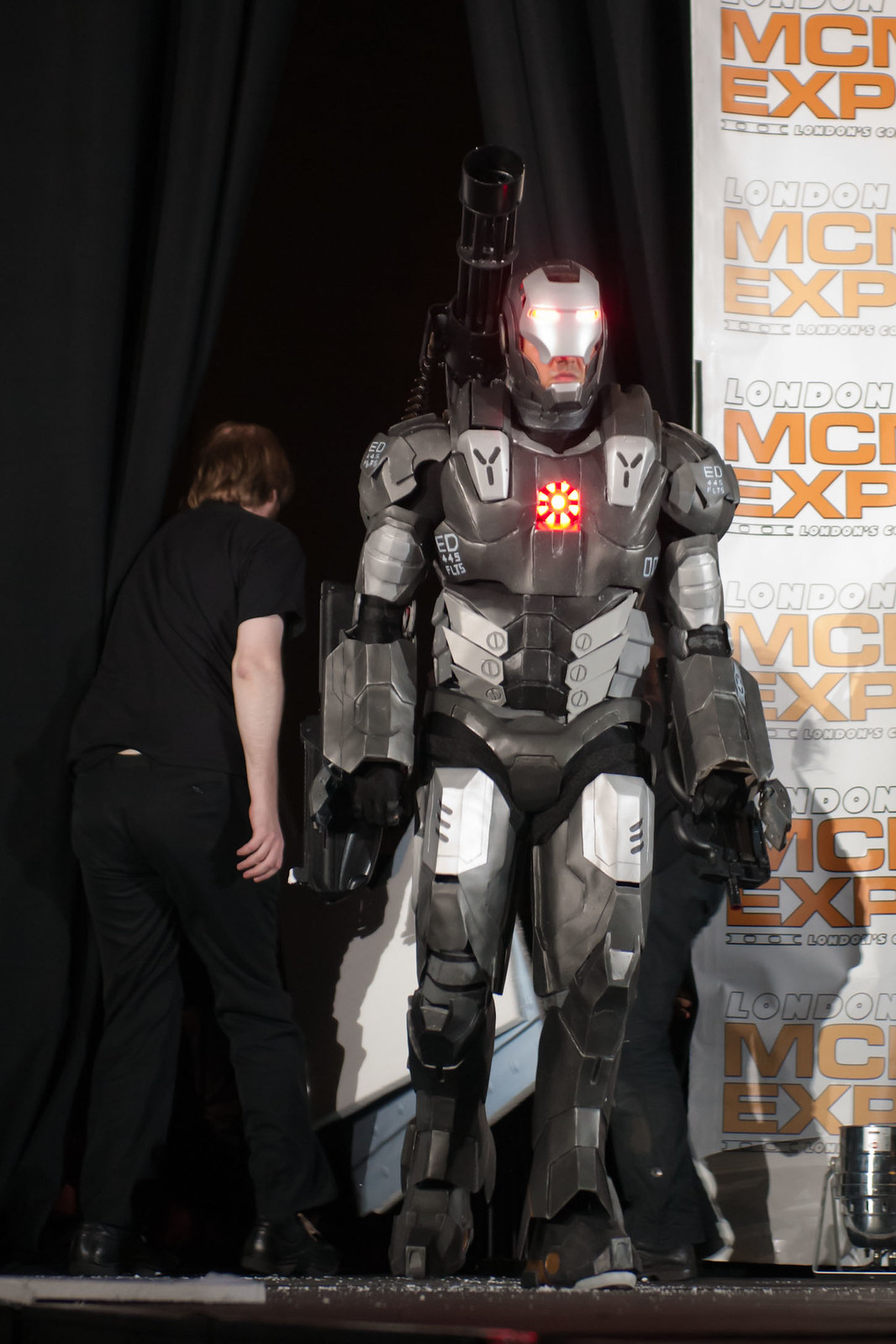This detailed photograph from the London MCM Expo London Comic Con showcases an impressive robot cosplay being presented on stage. The robot outfit, reminiscent of Robocop or Iron Man, features black and silver armor with illuminated eyes and a glowing circular emblem on its chest emitting yellow and red light. It also has a substantial laser cannon or weapon attached to its back. The robotic figure walks confidently towards the center of the stage in mechanized boots that add to its imposing presence. 

A large black curtain serves as a backdrop, with a tall white sign to the right proudly declaring "London MCM Expo." Behind the cosplaying figure, a white male with reddish hair is visible, dressed in a black t-shirt and black pants. He appears to be either controlling or assisting the robot, as he moves towards the curtain in the background, adding a touch of realism and intrigue to the scene. The vivid details, from the illuminated helmet to the fierce laser points, create an engaging and dynamic moment captured in this image.